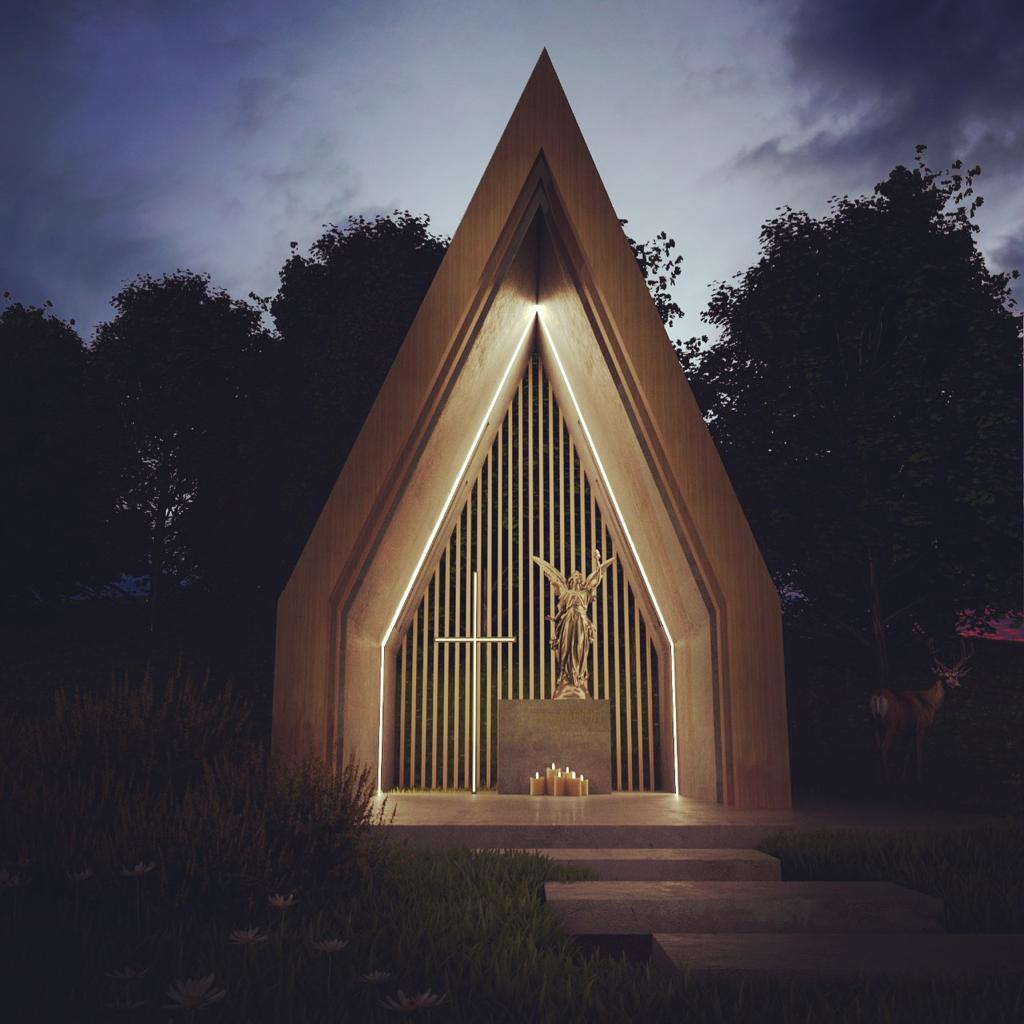In the middle of a secluded forest, this nighttime photograph captures a church-like memorial monument with a steep, pyramidal peak, made entirely of concrete. The structure is illuminated by LED lights, enhancing its austere beauty against a backdrop of dark, cloudy skies. Inside the monument, a cross is positioned on the left-hand side, while a golden angel statue stands majestically on a stone pedestal to the right. In front of the shrine, approximately six gold candles of varying heights cast a gentle glow. Surrounding the monument, a variegated stone pathway leads through the lush grass and foliage, guiding visitors towards the sacred space for contemplation and prayer. To the right, partially obscured by shadows, a stag with impressive antlers stands silently. The scene, framed by dense trees, combines the serene with the ethereal, creating an otherworldly, almost rendered appearance. The predominant hues of tan, gold, and green meld harmoniously to complete this tranquil sanctuary.